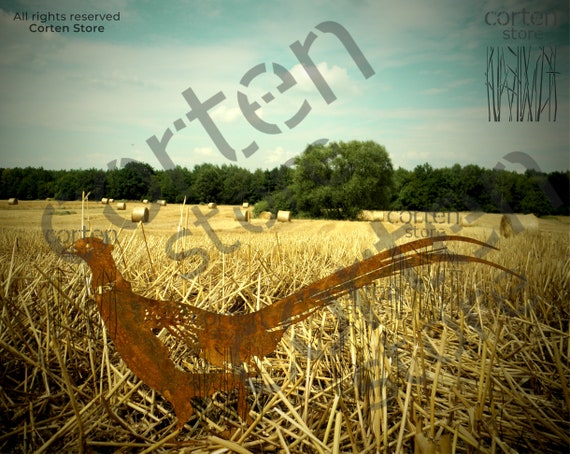The image captures a hauntingly picturesque scene reminiscent of a classic horror movie setting. It features a brown, sketch-like painting of a pheasant, which closely resembles a rooster, standing amidst a field of residual straw and dead grasses typical after a harvest. The ground is littered with scraps, adding to the eerie ambiance. Several large bales of hay are scattered in the background, set against a backdrop of lush green trees and a blue sky filled with clouds. In the top left corner, the text "All Rights Reserved, Corton Store" is prominently displayed, while "Corton Store" repeats in the top right corner and diagonally across the middle, similar to a watermark. The overall composition of the image, with its spooky bird and pastoral elements, creates a memorable and unsettling visual.